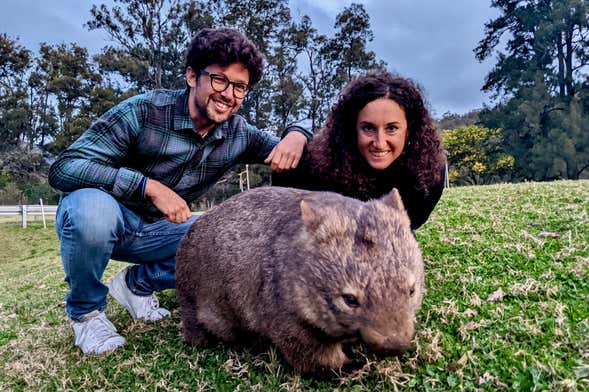In this outdoor daytime photograph, a kangaroo (or possibly a wallaby) is captured looking directly into the camera while munching on a sprig of green leaves. The animal's large, straight-standing ears are notably perked up. It has striking fur with a mix of colors—a dark brown overcoat with a contrasting white undercoat, including a distinctive white chest and patches of white that extend around its head and into its ears. The kangaroo's expressive brown eyes reflect a blue light, adding a captivating element to its gaze, complemented by a dark brown nose and slightly darker patches under its eyes. The background is out of focus but suggests a wooded area with varying vegetation, under natural daylight that hints at a clear blue sky. The overall ambiance suggests a tranquil outdoor setting.